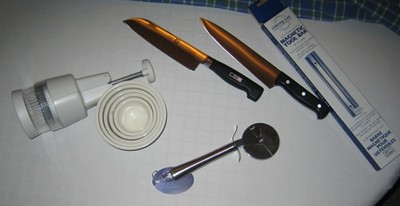This indoor color photograph showcases a collection of various kitchen utensils arranged on a white surface. In the upper right corner, two kitchen knives are prominently displayed—one being a cleaver and the other a chef's knife—both featuring black handles and gold-tinted blades. Next to the knives is a boxed magnetic toolbar, identifiable by its thin rectangular shape and blue printing, designed for mounting in a kitchen to securely hold the knives in place. Below the knives lies a stainless steel pie or pizza cutter with its blade oriented to the right and handle to the left.

In the lower left section of the photo, a white handheld chopper, possibly a Slap Chop, is positioned on its side with its plunger extending to the right and base to the left. To the right of the chopper, a set of nested white ramekins of various sizes can be seen. Additionally, there is a white handheld kitchen utensil, potentially a stirrer. Underneath this array of utensils, a white piece of fabric is draped over a blue plaid couch. All the items appear brand-new and unused, contributing to a clean and well-organized composition.